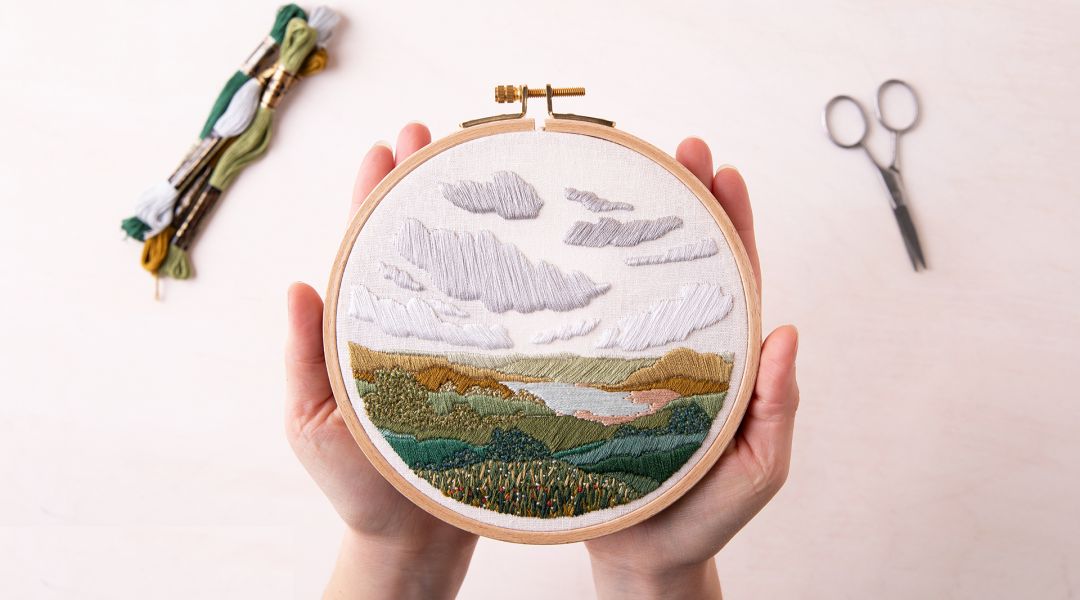The image depicts a handcrafted embroidery piece, likely created by a Caucasian woman, being held in both of her palms. The embroidery is a finished work, secured in a circular wooden hoop fastened with a screw at the top. The design on the fabric features a serene landscape; fluffy white clouds float in a blue sky above a meadow composed of green grass and hills, with a small lake nestled within. To the right of the embroidery piece, a pair of metal scissors points downward, while on the left side, four rolls of yarn in various shades of green, blue, yellow, and white lie bundled together. These elements rest on a smooth, light-colored surface, lending a gentle contrast to the embroidery focus which occupies the center of the image.